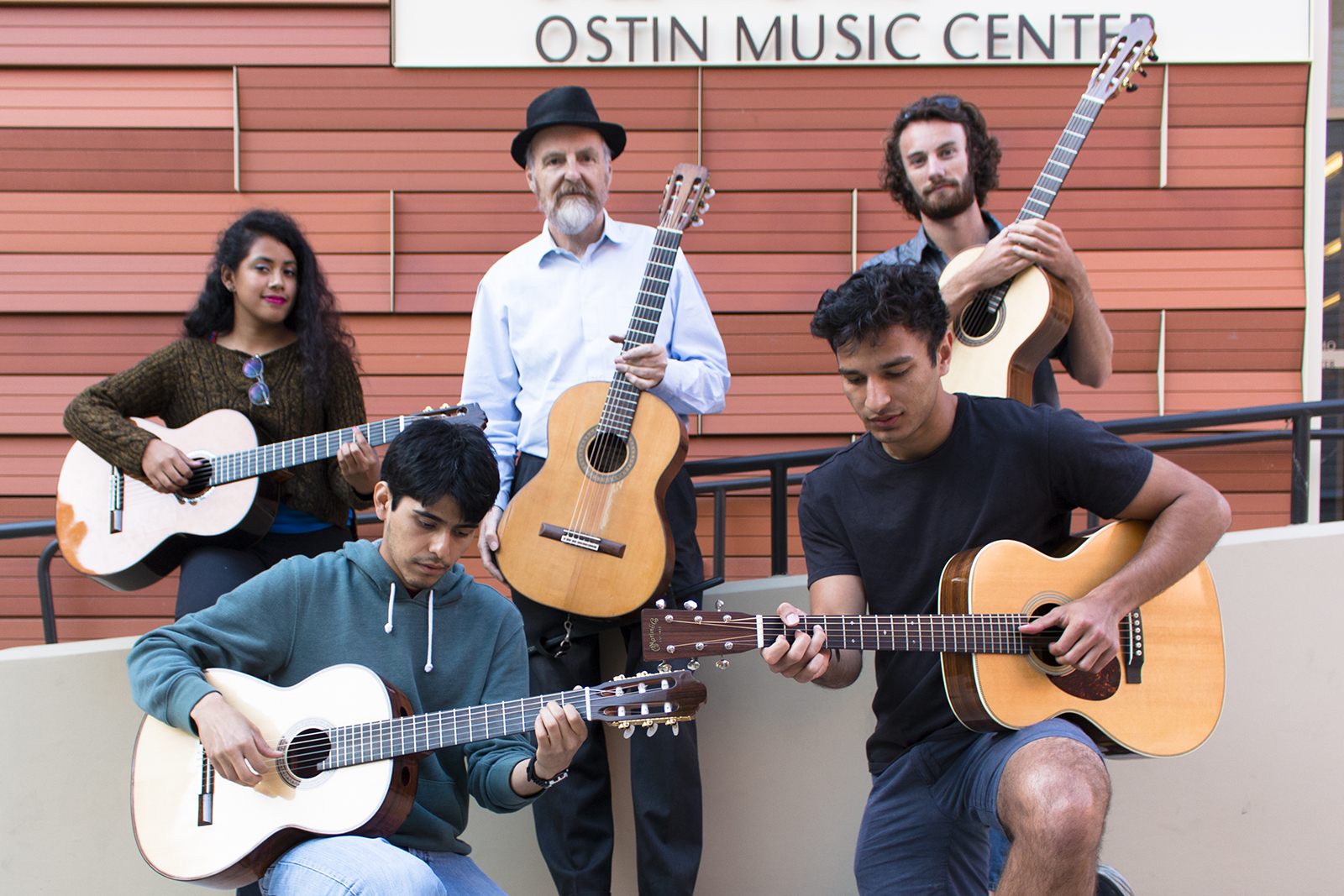This photograph captures a group of five individuals, four men and one woman, standing in front of a background featuring various shades of brown and red, possibly resembling aluminum siding. The prominent sign above them reads "OSTIN Music Center" in bold letters. 

In the back row, from left to right, stands a young woman with long curly black hair, wearing a green sweatshirt and blue jeans. She is holding a guitar, her glasses tucked into her shirt, and she is smiling warmly at the camera. Next to her is an older man, likely in his 60s, characterized by his black fedora, gray beard, and blue button-down shirt, holding his guitar upright with a composed demeanor. To his side, a tall man with long curly hair, a mustache, and a beard stands confidently, also holding his guitar upright and grinning at the camera. 

In front, kneeling, are two younger males. The one on the left, wearing a medium blue hoodie, holds his guitar as if he is about to strum it, focused on his instrument. Beside him, a young man in a navy blue t-shirt and shorts similarly holds his guitar and appears to be concentrating on it, directing his gaze downward. This assembly of guitar players radiates a sense of camaraderie and dedication to their craft, possibly with the older gentleman serving as their mentor or teacher.